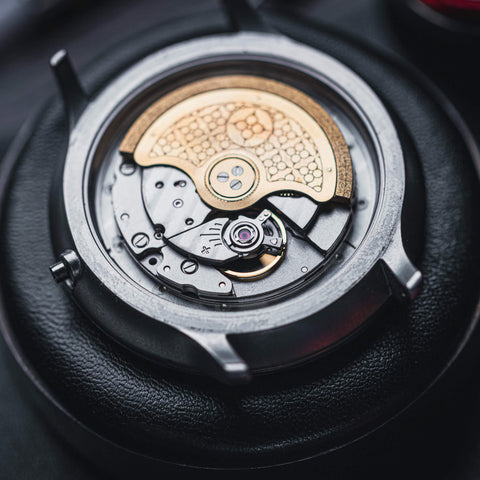This close-up photograph captures the intricate inner mechanisms of a disassembled watch. The silvery body of the watch, devoid of its band and back plate, is meticulously displayed on a plush, black, padded mat designed to prevent scratches. The watch’s circular frame is held securely in place by this cushioning. The highlight of the image is the exposed inner workings, showcasing several screws and dials. A striking copper-colored dial and what is likely the watch battery contrast with the predominant silvery components. A small silver button is visible on the left side, while band attachment points are identifiable on the upper and lower sections of the watch frame. A golden gear or half-circle shape adds a touch of contrast within the sophisticated, silvery sea of machinery, emphasizing the impressive engineering involved in the watch's construction. The photograph admirably captures the detailed and meticulous craftsmanship of this mechanical marvel.